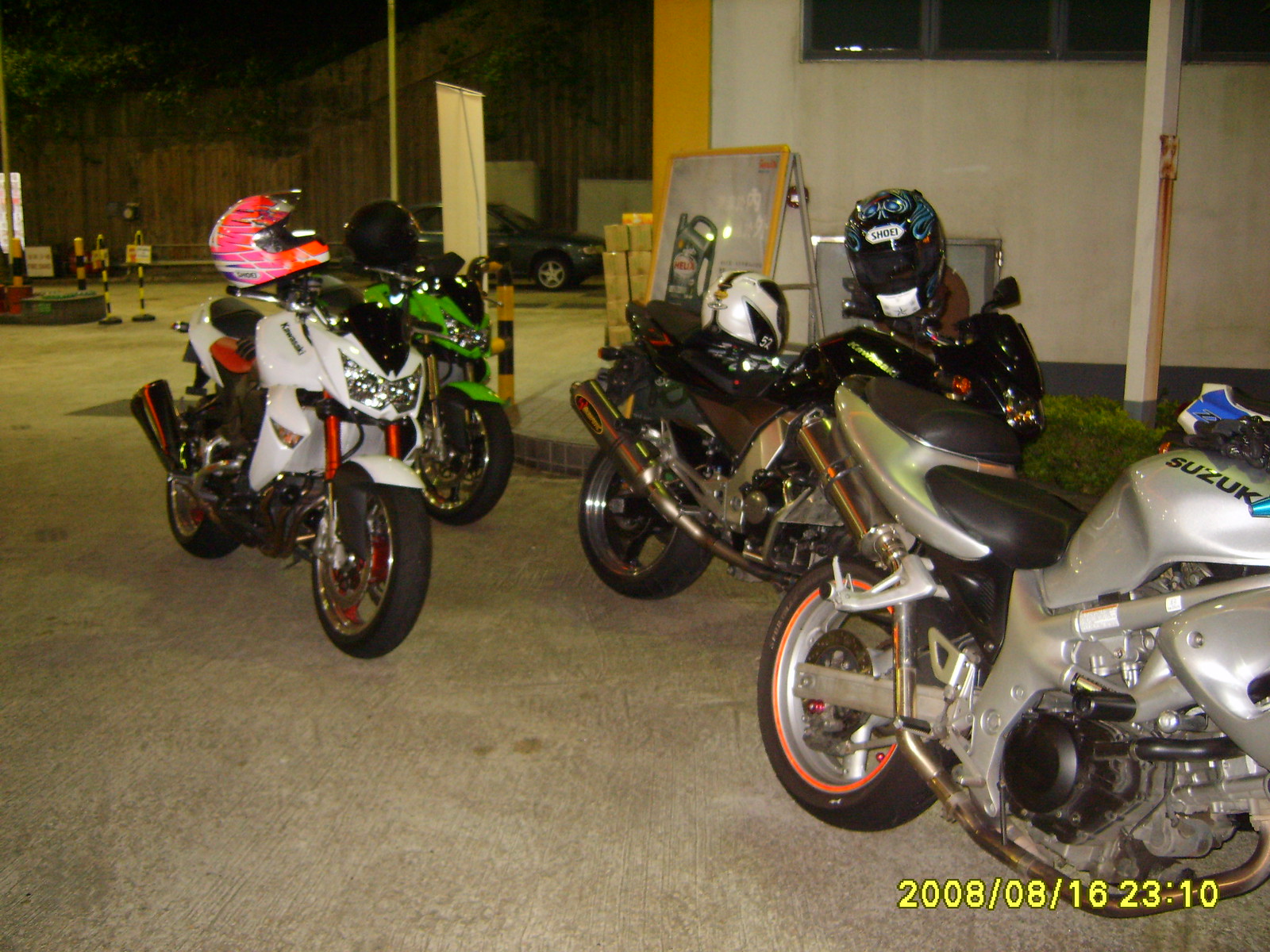This color photograph, taken on August 16, 2008, at 11:10 PM, depicts four motorcycles parked on a paved grey ground area, illuminated by artificial lighting from the upper left side. The scene is set in front of a nondescript white building with a yellow-edged window and a pole with illegible writing. 

Starting from the bottom right corner, the closest motorcycle to the photographer is a silver Suzuki. Behind it, there is a black motorcycle with multiple helmets placed on the seat and handlebars. 

To the left, a white motorcycle features black and red accents, and a pink, modern striped helmet is situated on its handlebars. In the back, a lime-green motorcycle with a black helmet, either on the handlebars or the seat, is partially visible.

Additional details include a stack of boxes on the sidewalk in front of the building and some temporary mobile posts on the left side of the image. Foliage and various signs are also visible in the background, giving context to the photo's setting. The date and time are superimposed in yellow text at the bottom right corner.